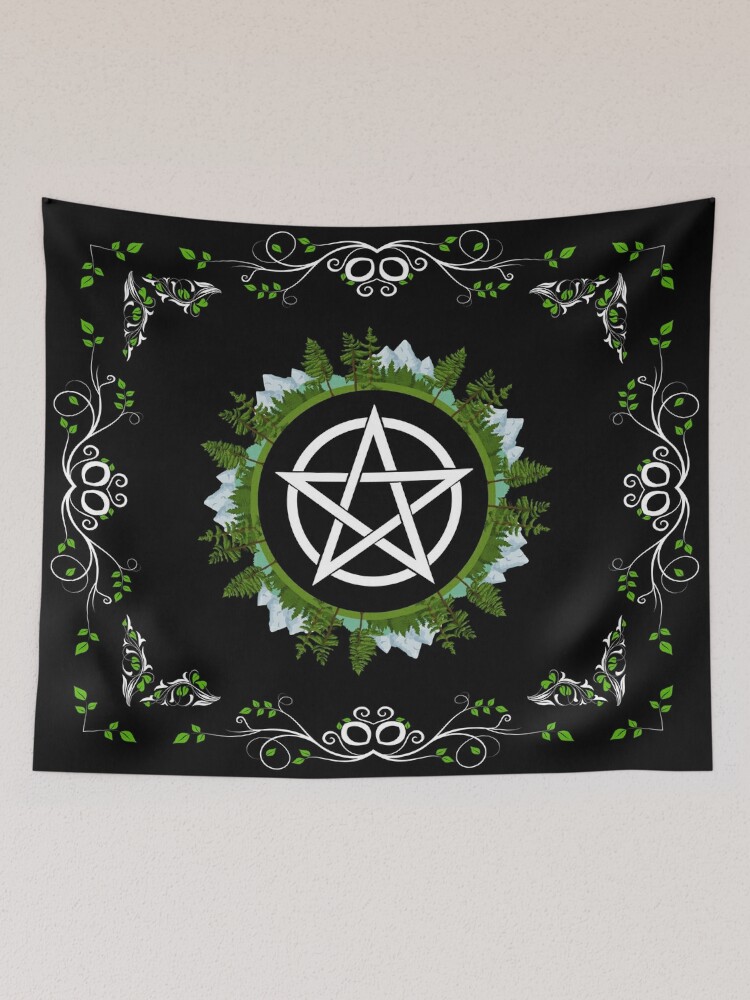This image displays a detailed, square wall hanging or tapestry set against a grayish pink background. The tapestry itself is entirely black, adorned with intricate white curly-Q decorations and vibrant green leaves that create a border around the edges. In the center of the tapestry, a prominent five-pointed white star or pentagram is enclosed by two concentric circles—a white inner circle and a green outer circle. Surrounding these circles are depictions of greenery, trees, and mountains, contributing to a sense of natural beauty and mysticism. The combination of floral elements and geometric symbols adds to the intricate and captivating design of the piece.